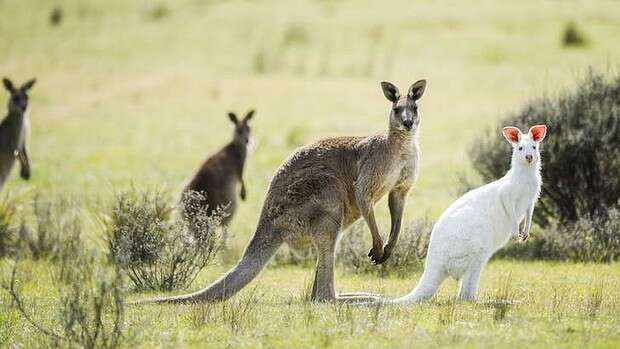The photograph captures a fascinating scene of four kangaroos in what appears to be a flat, dry, grassy field. Three of the kangaroos, all brown-tan in color, are positioned with their bodies facing right but their heads turned towards the viewer. The central kangaroo is in sharp focus, while two others in the background to the left remain slightly out of focus and blurry. Distinctly, on the right side of the image, stands a unique and highly noticeable albino kangaroo with white fur and pinkish ears, also in clear focus. Surrounding the kangaroos, the field is dotted with light green grass and scattered dry bushes, with one particularly large dark bush located behind the white kangaroo on its right side. The posture of the kangaroos, standing still on their hind legs, draws attention to their alertness, possibly reacting to the photographer’s presence. This image beautifully encapsulates a moment in the wild, showcasing the diversity among kangaroos in their natural habitat.